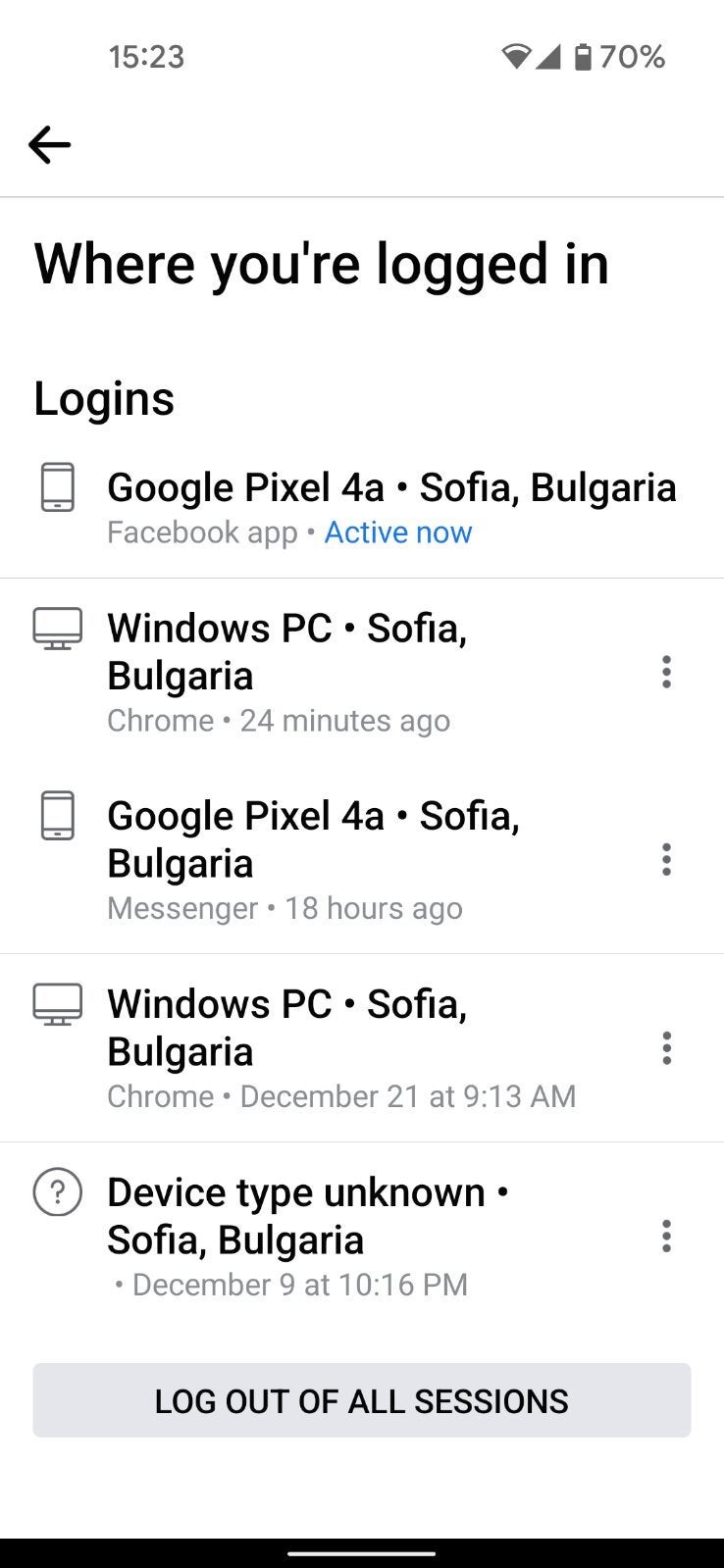The image presents a detailed overview of all active login sessions for a specific individual using various devices and browsers. Currently, the individual is logged in to the Facebook app on their Google Pixel 4a phone, located in an office in Safaya, Bulgaria. This session is active. 

24 minutes earlier, the user had logged in from the same office in Safaya, using a Windows PC with a Chrome browser. Additionally, there was a login session 18 hours ago from the same Google Pixel 4a phone in the same office. Another session is recorded on the 21st of December at 9:13 AM, during which the individual accessed Facebook via Chrome browser on a Windows PC, also from the office in Safaya, Bulgaria.

On the 9th of December at 10:16 PM, the individual logged in using an unidentified device type from the same office location. At the bottom of the screenshot, there is a grey rectangular button labeled "Log out of all sessions," indicating the option to terminate all active sessions across these various devices and browsers if necessary. The application effectively tracks and displays the login history, providing an option to manage session security.